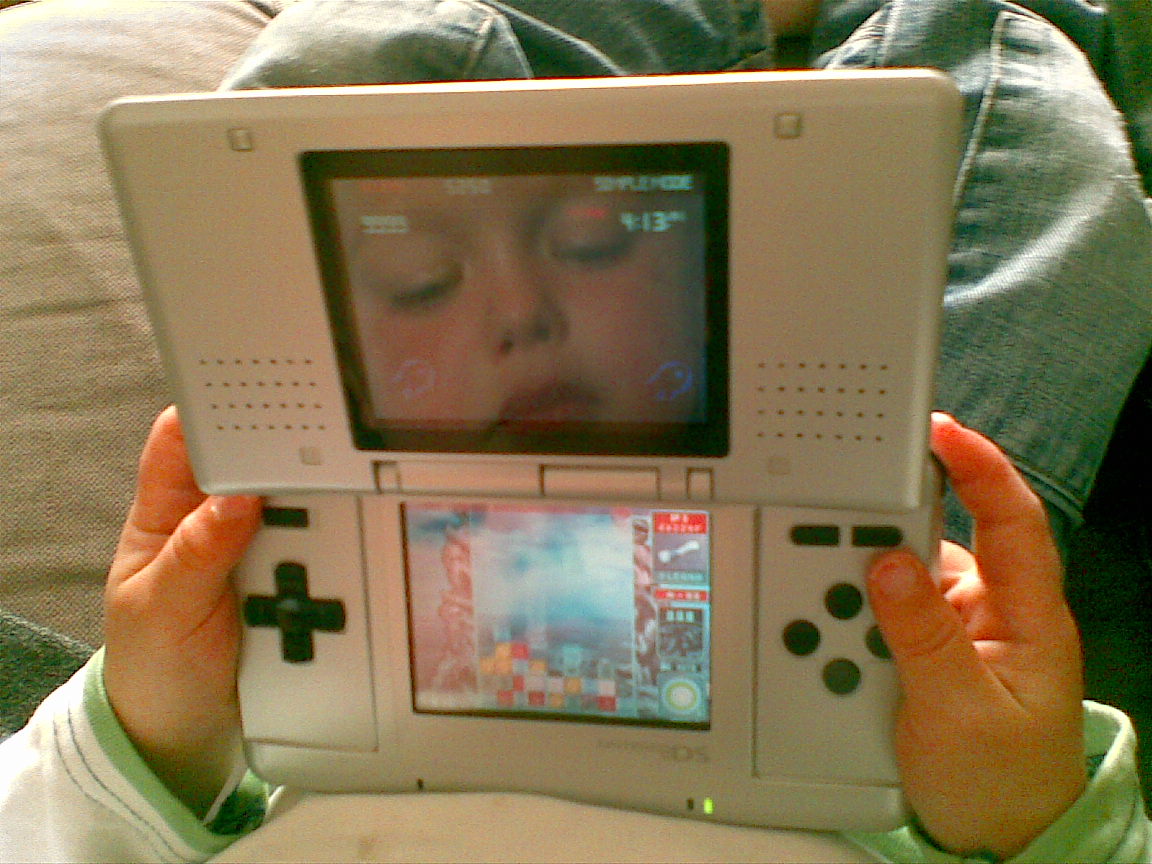The photograph depicts a child, with small hands likely belonging to a toddler or young child, engaging with a Nintendo DS handheld game system. The child is wearing a long-sleeved white shirt with green bands at the wrists. The DS system is white with black buttons and features two screens. The top screen displays a reflection of the child’s face, showing a neutral expression and also displaying the time "4:13" alongside some indistinguishable text. The bottom screen shows a blurry game in progress, making it difficult to identify the game. A small green light and the partially readable letters "OS" are visible at the bottom of the gaming device. The child appears to be sitting on a light brown surface, dressed in faded blue jeans.